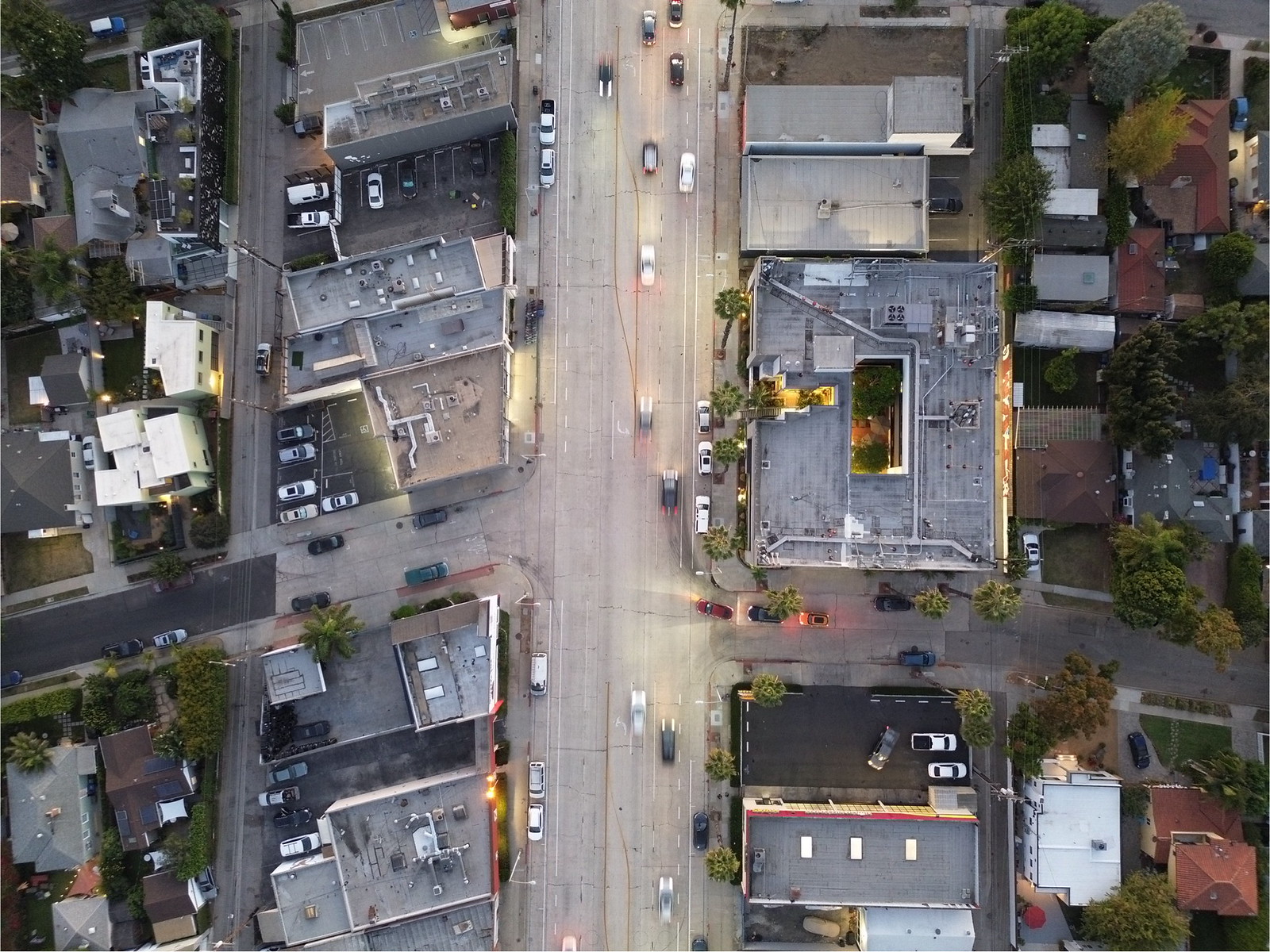The aerial photograph captures a wide, divided roadway cutting through what appears to be a bustling California city. The scene is bathed in sunlight, highlighting the distinctive rows of palm trees lining the broad road. The main thoroughfare, featuring a concrete median, boasts three lanes of traffic in each direction, with one possibly designated as a parking lane.

Radiating out from this central artery, smaller roads branch off at various angles. On the left side of the image, a narrower, two-to-four-lane road runs parallel to the main road, bordered by numerous commercial buildings. These structures, characterized by flat roofs and visible air handlers, suggest a business district. Interspersed among them are parking lots, some with only a handful of cars, indicating moderate activity.

A wedge-shaped building and its adjacent parking area, housing about five cars, nestle into one of the angled corners. Further along, another elongated structure with a flat roof presides over a larger parking lot, accommodating roughly half a dozen vehicles.

Traffic on the main road appears light, with approximately 20 cars visible. On the right side, the sun's rays reflect off several buildings, adding a dynamic play of light and shadow to the scene. Behind the commercial buildings, residential areas begin to emerge. These neighborhoods, marked by smaller homes with peaked roofs and visible lawns, suggest a tranquil retreat from the bustling main road. Similar residential zones can be seen one block behind the businesses on the left side, creating a clear transition from commercial to residential spaces within the cityscape.